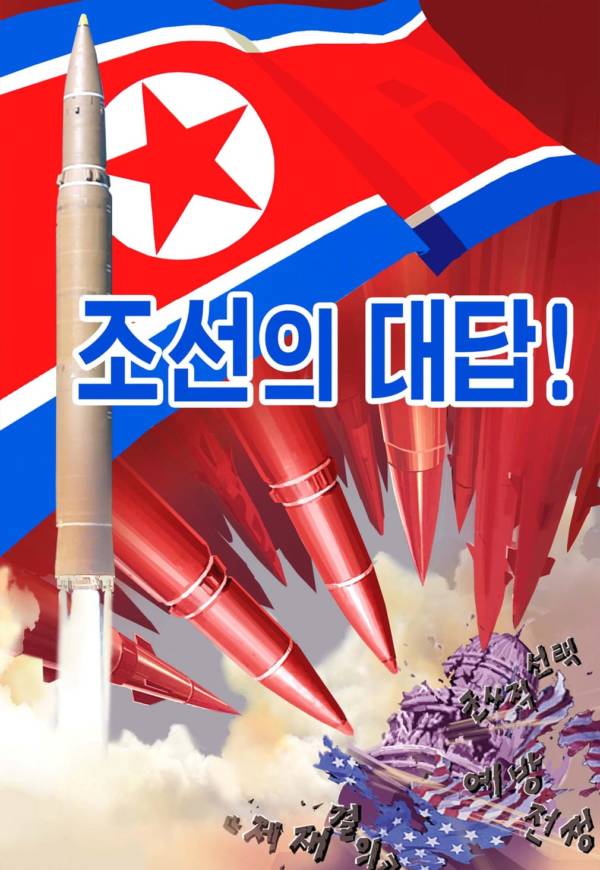The image depicts a vivid, propaganda-style artwork reminiscent of old wartime posters. Dominating the top of the image is the North Korean flag, characterized by its bold red color, white circle, and a prominent red star, flanked by blue and white stripes on the sides. Below the flag, several red missiles are ominously pointing downward towards the U.S. Capitol building in the bottom right corner, which is depicted in ruins, indicative of an assault. Adding to the scene’s chaotic atmosphere, an American flag is visible, torn and tattered. The backdrop features a gray sky filled with billowing clouds, emphasizing the destruction. A single gray missile ascends diagonally from the bottom left to the top left of the image, leaving a fiery trail behind it. The entire composition is accompanied by bold, 3D black Asian characters above the scene, likely a political slogan, rendered in a graphic style font. This compelling image combines elements of traditional propaganda with comic book artistry to evoke a strong message of conflict.